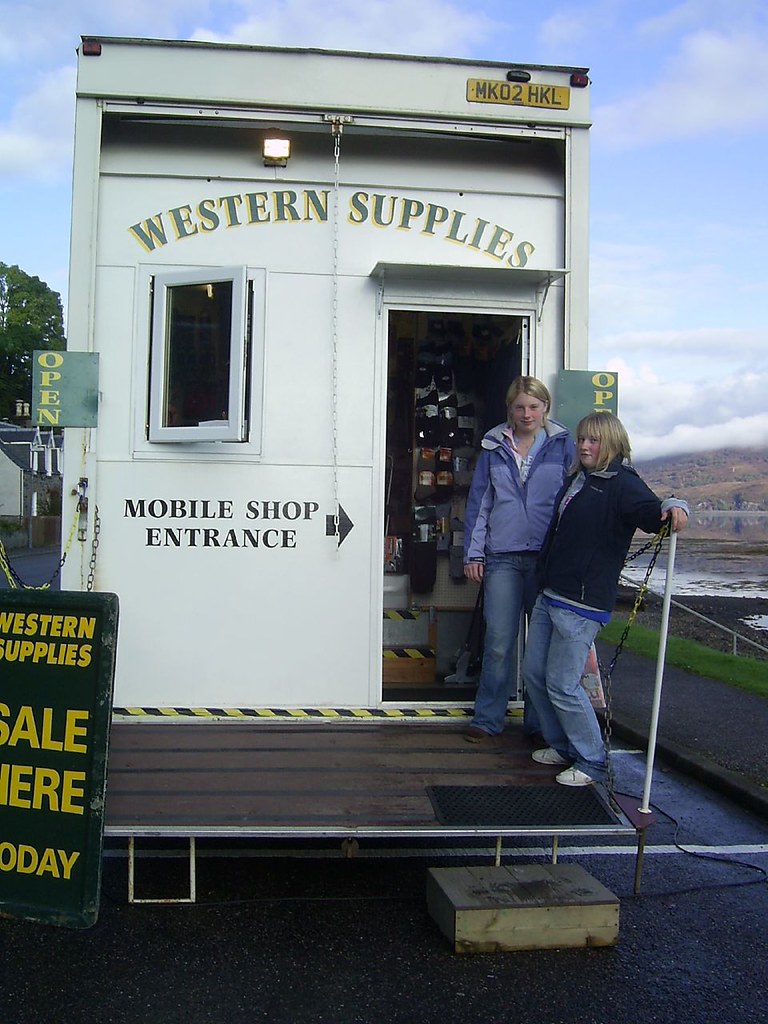This image depicts a close-up view of a truck functioning as a mobile shop, adorned with the name "Western Supplies." The back of the truck is visible, showcasing a small, arch-shaped doorway with the words "Western Supplies" displayed in green above it. To the left of this doorway, there's a little window, and adjacent to it, a sign pointing to the entrance that reads "Mobile Shop Entrance." On either side of the entrance, green squares with "Open" written in yellow letters are visible. The truck also features a prominent sign in front that states, "Western Supplies, Sale."

Within the open doorway, various items for sale are displayed. In front of this entrance, two blonde teenage girls stand. One girl is dressed in a purple jacket paired with blue jeans, while the other sports a black jacket, blue jeans, and white shoes. The background reveals a landscape with mountains and a lake on one side, and some buildings and a tree on the other, adding to the scene's rustic charm.